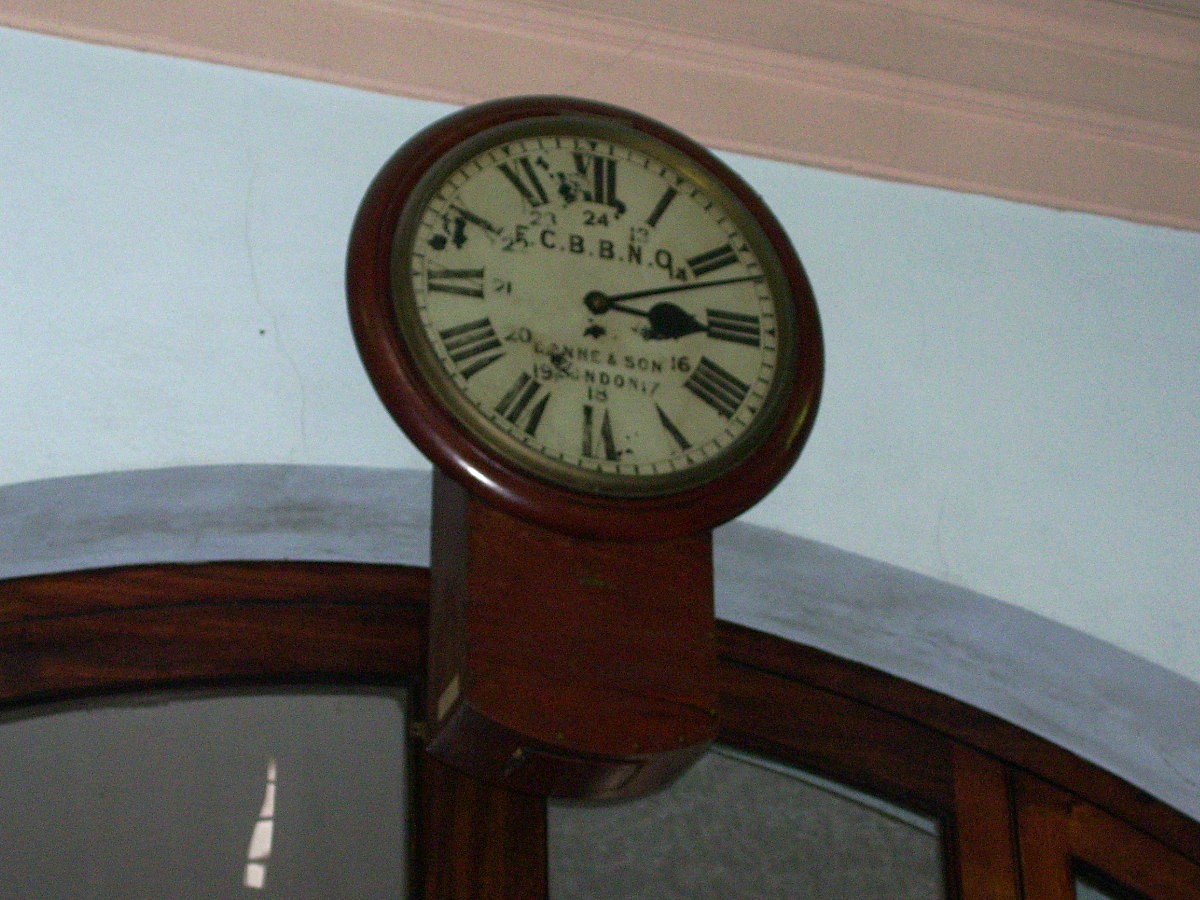A vintage-style clock captured from a low angle, showcasing its dark cherry wood frame, which exhibits subtle lines and textures indicative of its age. Encircling the clock face is a fine gold ring that contrasts elegantly with the white background of the clock. The clock features black hour and minute hands, along with Roman numerals marking the hours. The time displayed is 3:12. Additional details on the clock include the letters "C-B-B-N-O" and a partially faded word beneath them, hinting at the passage of time. The clock is mounted on a large piece of furniture, also crafted from the same rich cherry wood, though only a part of this furniture is visible in the image.